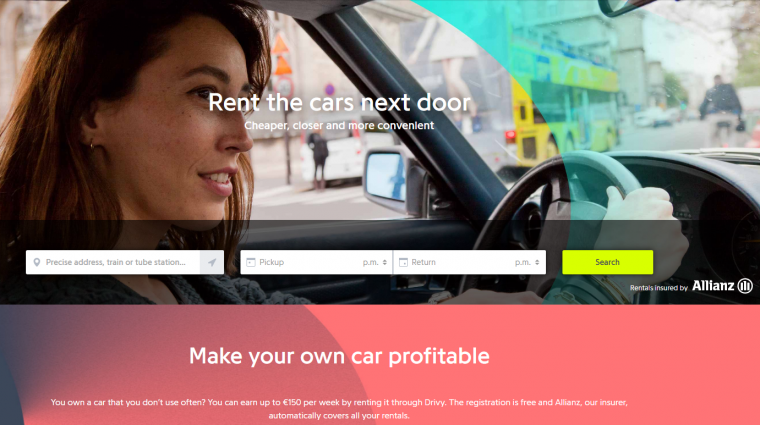**Detailed Caption:**

The image is a promotional advertisement for a car rental service, as depicted in the screenshot. The focal point of the advertisement is a woman sitting inside a vehicle, looking to her right. She appears to be in her 30s, with dark brown hair and a single earring visible. Her mouth is open in a neutral expression, neither smiling nor frowning, and her brown eyes are looking towards something outside the car. Her hands rest on the steering wheel.

The background of the image is blurred, showing indistinct shapes of cars, buses, and people, suggesting a busy road scene. Overlaid on this image, near the woman’s eyes, is the text "Rent the cars next door" in white. Below this, the caption reads "Cheaper, closer, and more convenient."

At the bottom of the advertisement, aligned centrally, are three search boxes labeled "Precise address, train or tube station," "Pick up," and "Return." Adjacent to these boxes is a neon greenish-yellow search button with the word "Search" in black text. To the right of this button, in the same green color, is the text "Renters insured by Alliance," accompanied by a logo.

The bottom section of the advertisement features a red background with white text. It includes a call to action: "Make your own car profitable." Below this message, additional details are provided: "Do you own a car that you don't use often? You can earn up to 150 British Pounds per week by renting it through Drivee. Registration is free, and Alliance, our insurer, automatically covers all your rentals."

This detailed caption aims to describe the advertisement comprehensively, highlighting its visual elements, text, and overall layout.